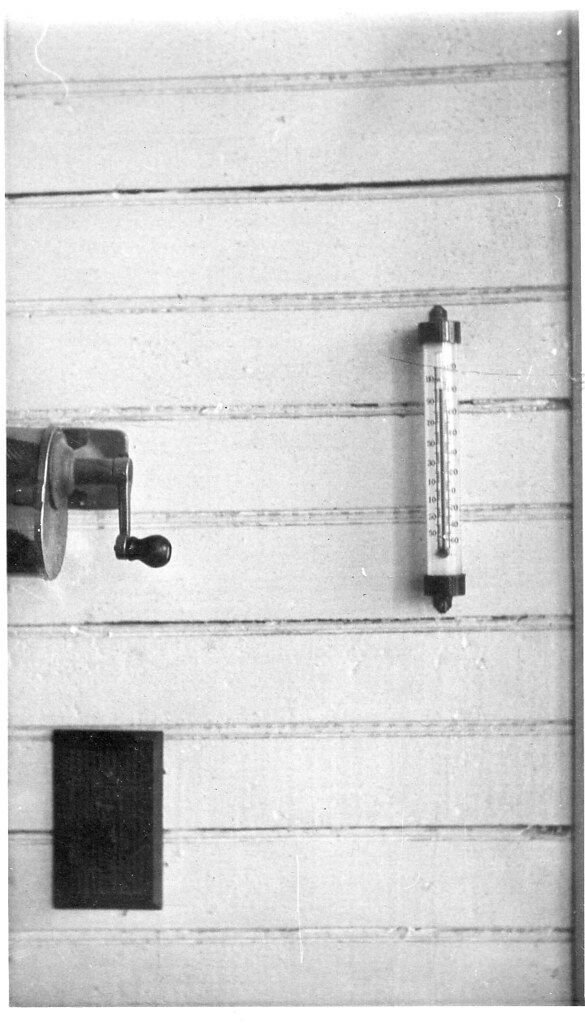The image depicts a section of a white beadboard wall, featuring a few distinct elements. On the right-hand side, there is an old-fashioned thermometer with a white tube displaying black numbers and hash marks. A visible line runs up the center of the tube, and the top and bottom are capped with black, likely plastic, end caps. To the left of the thermometer, extending off the page, is a crank mechanism that appears to be part of a metal paper towel holder. Below this assembly, there is a power outlet with a black cover and black outlets. The image, likely a black-and-white photograph, showcases nine vertical slats of the beadboard paneling.